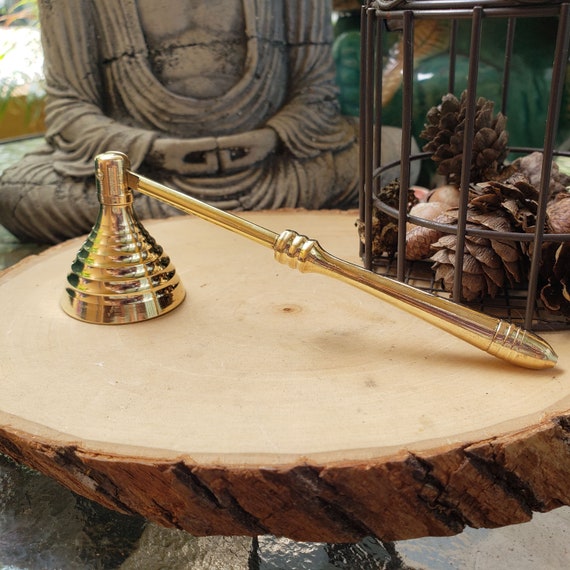In this detailed color photo, we're presented with an intriguing scene set on a rustic table crafted from a slice of a tree trunk, featuring a brown outer bark layer and a light-colored wooden center. Dominating the scene is a peculiar device resembling a candle snuffer, adorned in a gold hue with ridges along its horizontal handle that terminates in a cup-like end, suggesting it could be used to extinguish flames. Adjacent to this device is an open, wire-framed basket filled with brown pine cones and scattered leaves, resembling a small bird cage. In the background, partially visible from the chest down, stands a grey Buddha statue with a serene presence. The statue depicts a robed figure with hands positioned in a meditative gesture, fingers and thumbs touching. The setting appears to be either outdoors or very close to an outdoor space, as suggested by the abundant natural light and glimpses of greenery, adding a tranquil, nature-infused ambiance to the scene.